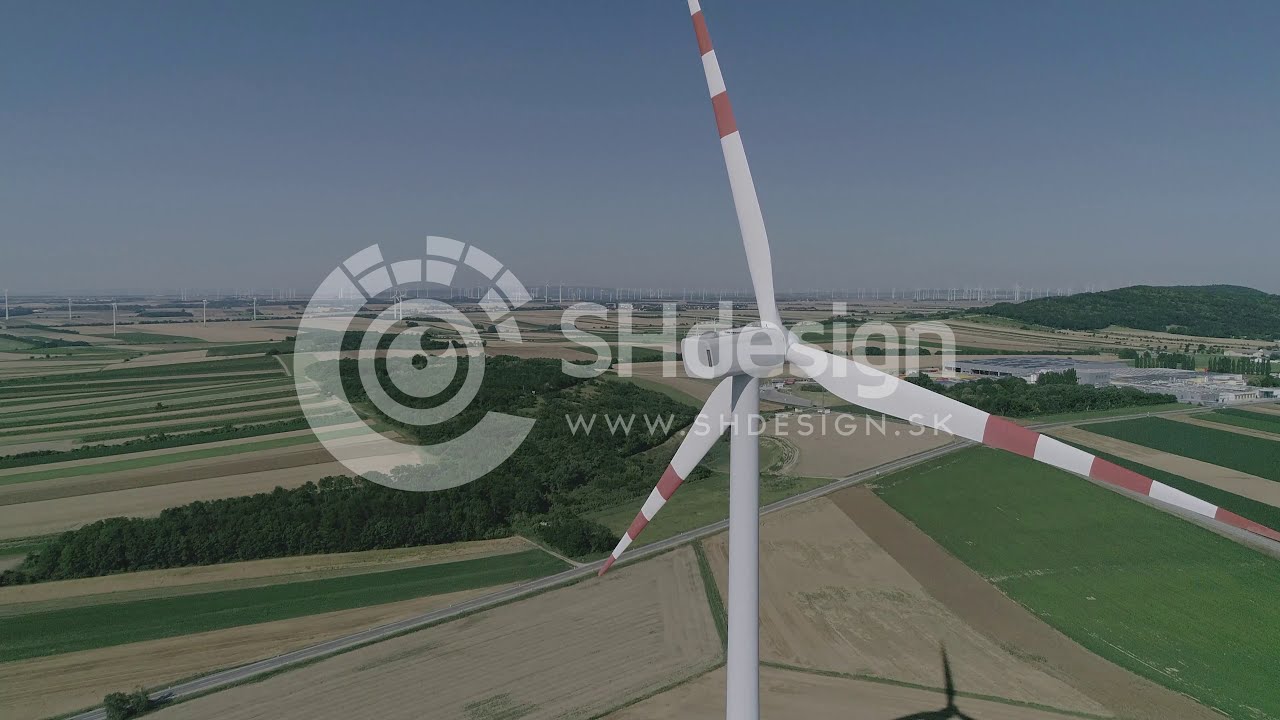The image is a highly detailed, photorealistic view from above of a white wind turbine positioned just right of center. The turbine, featuring three blades, dominates the image, with one blade intersecting the top, one the right side, and one pointing downward to the left. Each blade has three red bands spaced evenly along its length. The turbine casts a shadow to the bottom right, suggesting sunlight from the left.

The background displays a patchwork of meticulously maintained fields in alternating shades of dark green and light brown, akin to various stages of crop growth or types of vegetation. Trees punctuate the landscape, while a large, densely vegetated hill rises on the right. Multiple smaller white wind turbines dot the distant fields.

The sky forms the upper third of the image, transitioning from a darker blue above to a lighter blue near the horizon. Embedded in the center of the image is semi-transparent white text reading "SHdesign," with smaller text below that reads "www.shdesign.sk." To the left of the text, a logo resembling a large 'C' encircling two small circles is visible.